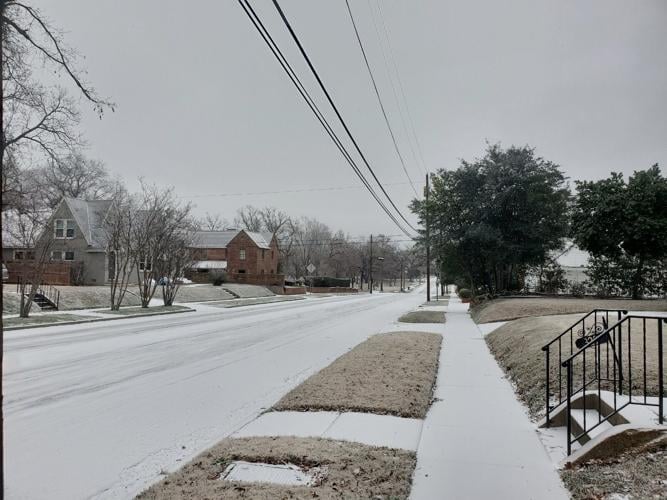This image depicts a quiet, snow-dusted town street in Anytown, USA. The scene is taken from a sidewalk that extends straight into the distance, running parallel to a two-lane road, both covered by a thin layer of snow. In between the sidewalk and the road are evenly spaced power lines. 

On the left side of the image, two-story houses sit atop small embankments, connected to the sidewalk by cement pathways and steps, all lightly covered in snow. The trees lining this side of the street are bare, typical of winter, although in the background to the right, evergreen trees add some green to the otherwise muted palette of whites, grays, and faded browns. You can see telephone poles and wires stretching across the top of the image.

The road is icy and untouched by traffic or pedestrians, enhancing the serene, almost desolate atmosphere. The houses, stairs, and trees all display a delicate layer of snow, contributing to the overall wintery feel of the scene.